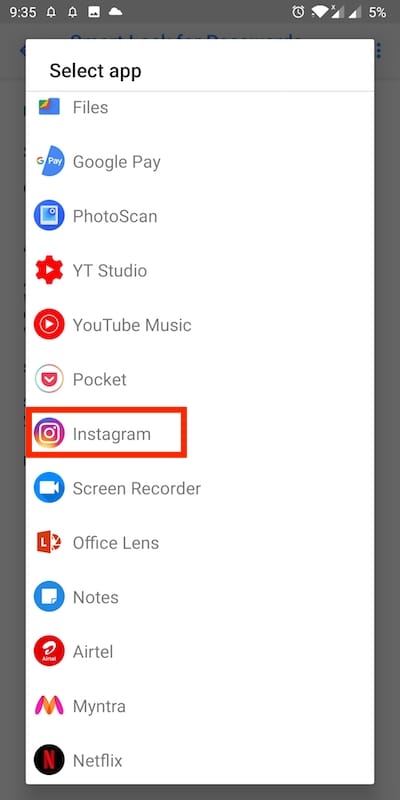This image appears to be a screenshot taken from a smartphone, judging by its narrow vertical dimensions and the presence of typical phone UI elements at the top. These elements include icons for the current time, alerts, battery percentage, and Wi-Fi connectivity. Below these symbols, a header in bold text reads "Select App," indicating that the user is in the process of choosing an application from a list.

The main content of the screenshot showcases a scrollable list of approximately a dozen applications, each represented by its respective icon on the left. Among the apps visible are Files, Google Pay, Photoscan, YouTube Studio, YouTube Music, Pocket, Instagram, Screen Recorder, Office Lens, Notes, Airtel, Myntra, and Netflix. Notably, the Instagram app stands out prominently, as it is enclosed in a thick red box, suggesting that it has been selected or highlighted for some reason, whereas the other apps are listed in a standard format.